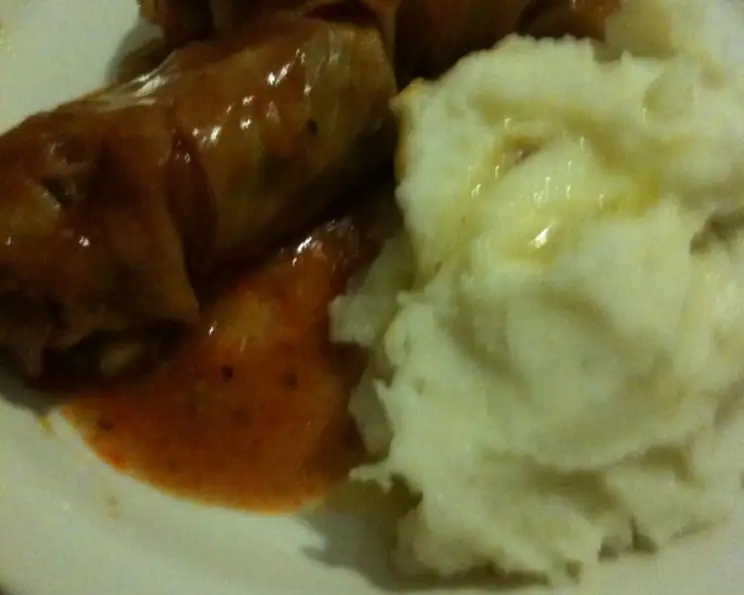This image shows a very close-up, somewhat blurry photograph of a meal on a white plate. On the right side, there is a serving of mashed potatoes, which appear white and fluffy with melted butter on top. On the left side, there is a log-shaped item that could be a dolmus (stuffed fig leaf), a sausage, or some other kind of meat or wrapped food. It is covered in a thin, tomato-y or brownish gravy, some of which is also splattered on the plate between the mashed potatoes and the log-shaped item. The image lacks any text or additional context, and its extreme zoom creates a fuzzy resolution, making it difficult to discern finer details.